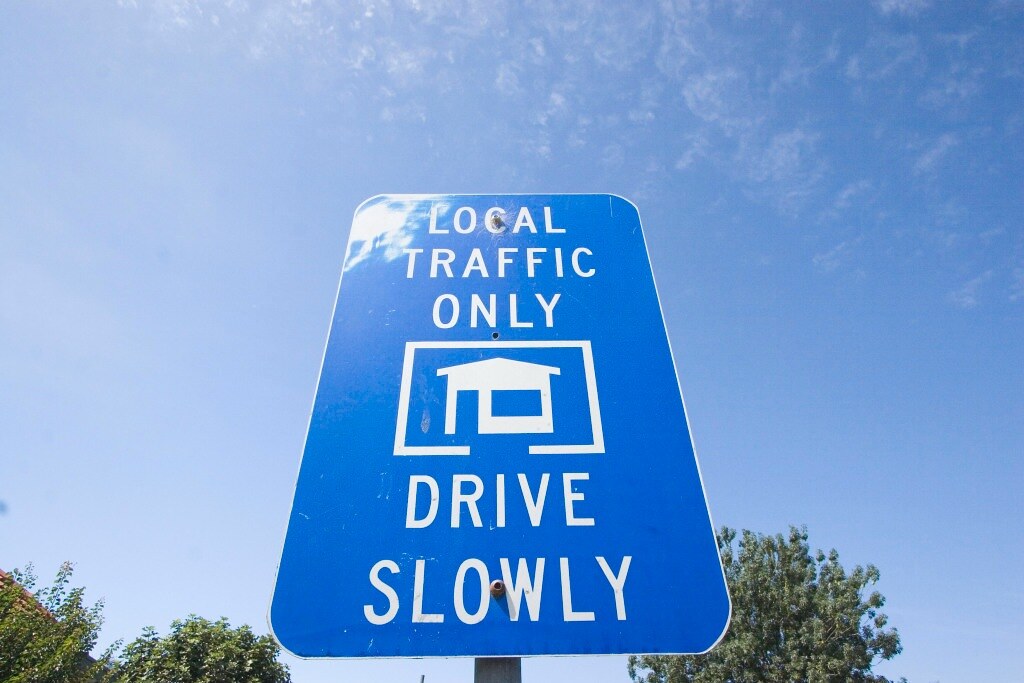The photograph captures an upward-angled view of a traffic sign against a light, clear blue sky, adorned with a few wispy white clouds. The sign is prominently dark blue with a white border, and it bears the inscriptions "Local Traffic Only" and "Drive Slowly" in clear white print. Centrally, it features an illustration of a house with a door and window, encased in a rectangle open at the bottom. Lush greenery and leafy trees create a verdant background, while the metal pole supporting the sign is visible. A gray metal bolt affixes the sign to the pole, conspicuously situated between the "O" and "W" in "slowly". The sun's light reflects off the top left corner of the sign, causing a subtle distortion.